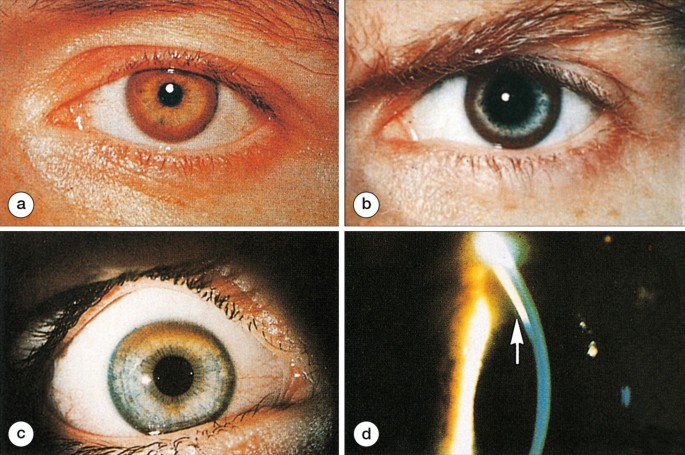The image is a rectangular collage longer than it is wide, divided evenly into four quadrants by white lines, forming a plus sign layout. Each quadrant is labeled with a white circle outline containing a respective letter: A, B, C, or D.

- **Top Left (A):** Depicts a close-up of a brown eye. The surrounding eyelids and eyebrow exhibit noticeable redness, hinting at irritation. The gaze is directed straight at the lens, suggesting a neutral or slightly focused expression.
  
- **Top Right (B):** Shows a very dark eye, almost black, with a slight presence of redness in the corners. The eyebrow appears furrowed, contributing to an angry or intense appearance. The iris features a dark brown hue with intricate detailing.

- **Bottom Left (C):** Features a close-up of an eye with a complex coloration. The pupil is black, surrounded by light brown, which transitions into a strikingly light blue iris. There are hints of light brown at the very bottom of the iris. The eye is framed by dark, prominent eyelashes, and the background is black, enhancing the eye's vivid hues.

- **Bottom Right (D):** Breaks from the eye motif with a different image entirely. It shows a black background with a central object resembling a blue table lamp. A bright white and yellow line descends from this, and there are two fibrous structures pointing upwards with differing color patterns—one green, blue, and white, and the other orange, brown, and white. Dots in blue, white, brown, and light brown are also present to the right of these structures, along with a white arrow pointing upwards, rendering the image ambiguous and open to interpretation.

This detailed description encapsulates the prominent features and nuances from each captured perspective.